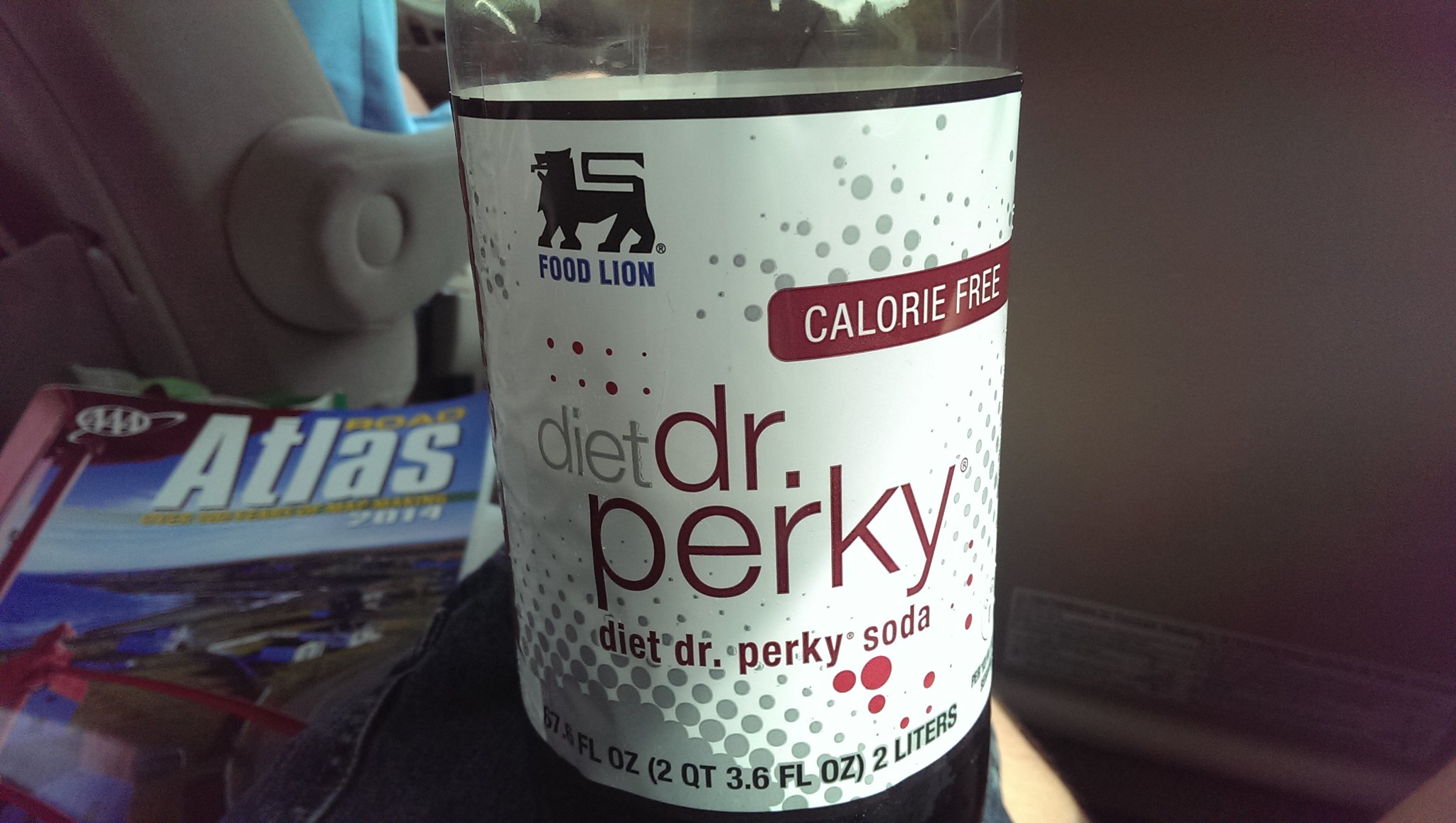This detailed photo, taken from the back seat of a car, focuses on a half-empty bottle of Diet Dr. Perky soda, the Food Lion store brand. The bottle, prominently displaying a white label adorned with small gray and red dots, lists "calorie-free" in a red background with white letters. "Diet Dr. Perky" is written twice in red letters on the label, and it indicates a volume of 2 quarts, 3.6 fluid ounces, or 2 liters. To the left of the bottle rests a blue AAA 2014 Road Atlas, featuring a beach scene with water on its cover. Behind the atlas, a person in the driver’s seat is seen wearing a light blue shirt, and the car seats are grayish-brown. The back of the passenger seat is visible in the upper right section of the image, while a blue jean pant leg is discernible beneath the bottle, underlining the casual and lived-in atmosphere of the car’s interior.